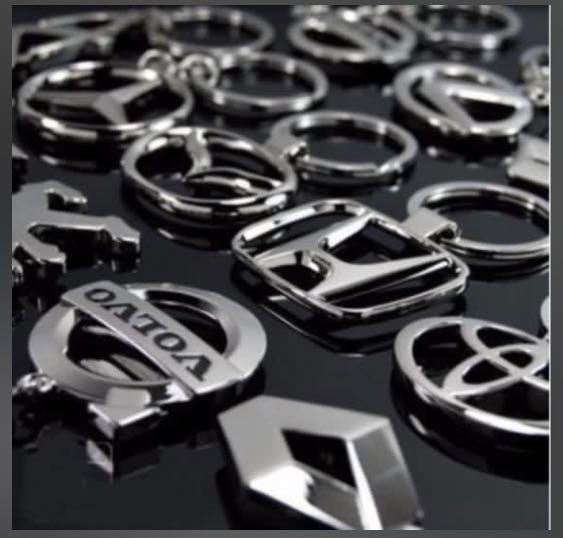The image showcases a collection of silver car manufacturer emblems attached to keychains, artfully arranged on a glossy black surface that resembles the sheen of a car hood. Prominently positioned in the bottom left is the Volvo emblem, albeit upside down. Moving upwards, there is a distinct Toyota emblem featuring its iconic triple ovals, followed by Honda's recognizable "H" within an oblong square. Adjacent to Honda is Mazda with its sleek wing-like symbol, and next to it, the Mercedes-Benz three-pointed star. Other visible emblems include Hyundai and Ford, although some in the background are blurry and indistinct. All emblems are roughly two inches in length and are equipped with small keyrings at the top.